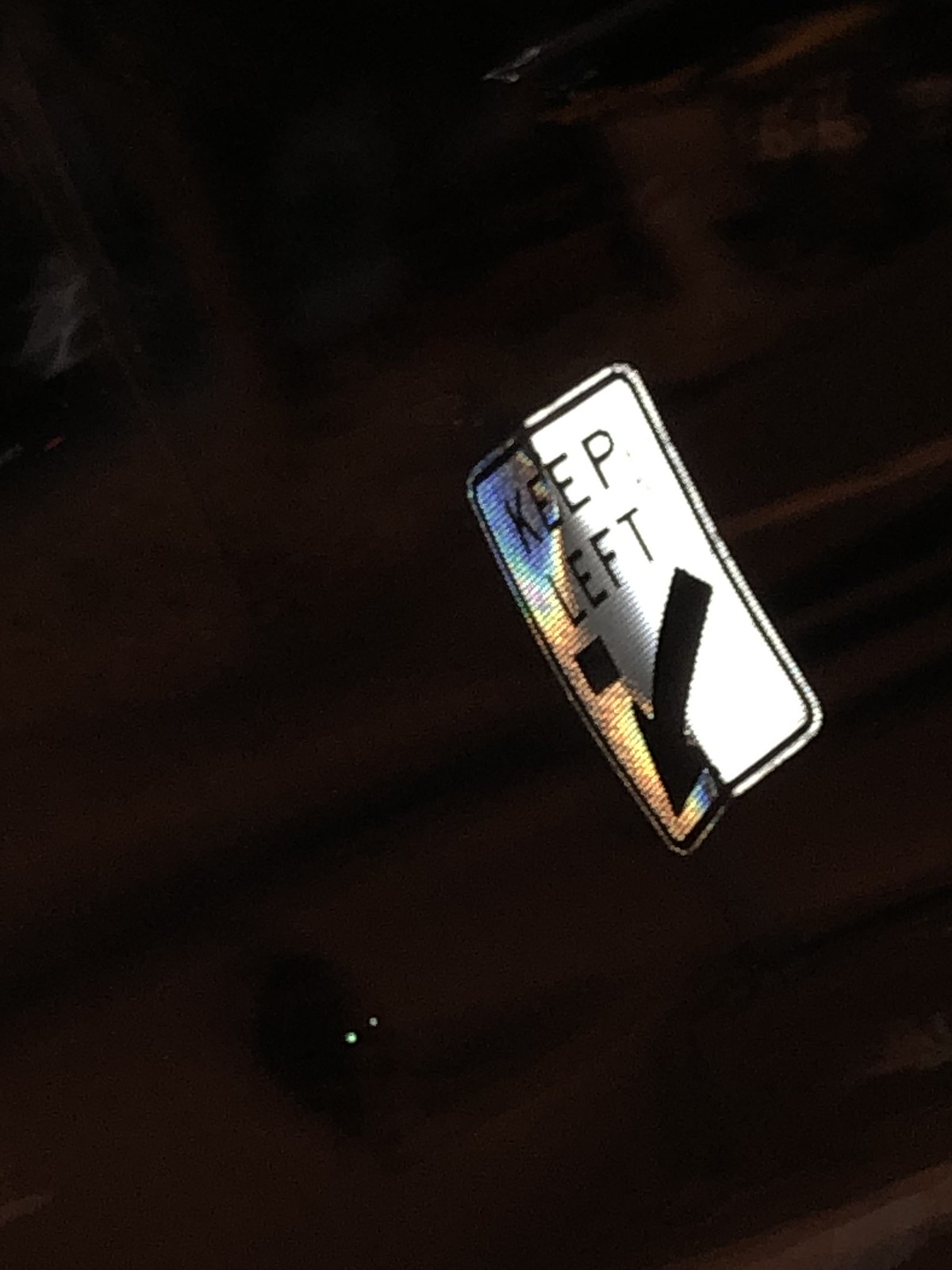In this nighttime photograph, a bent street sign is prominently featured, appearing to have suffered an impact that has left it leaning at an angle. The rectangular sign, with a white background and bordered by a black line, bears the message "Keep Left" in bold black text, accompanied by an arrow pointing diagonally to the bottom left. The reflective nature of the sign causes its right side to shine brightly white under the illumination, while the left side reflects hues of blue, orange, and yellow. The scene is somewhat distorted, possibly indicating the photo was taken at a high speed or from an unusual angle. The dark backdrop of the image is punctuated by the eerie presence of glowing eyes at the bottom left, belonging to a dark, indistinct creature that might be wildlife or a dog. Additionally, the upper half of the image shows a blurry outline of a large, leafless tree to the left side, adding to the night's mysterious atmosphere.